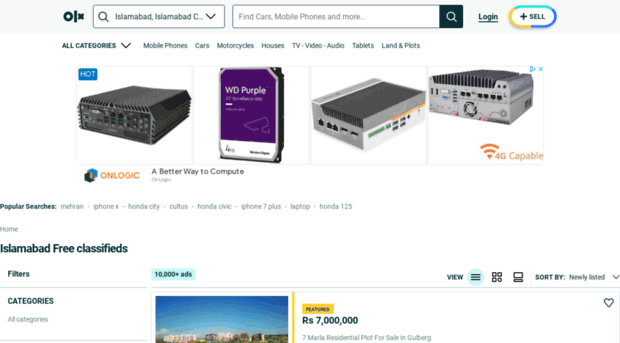This image features a storefront webpage, presumably based in Islamabad, as indicated by the text in the search bar and various elements throughout the page. The currency is listed as Rs, which suggests it could be Pakistani Rupees, based on the geographic context. The main section is populated with images of networking and server equipment. Prominently, there is a black device adorned with multiple ports and labeled as 4G capable, indicative of enterprise networking gear capable of generating wireless signals. Adjacent to this, another noteworthy item is a large Western Digital (WD) Purple mechanical hard drive, often used in server settings due to its sturdy construction and high capacity.

The top of the page features a navigation bar with a central search bar pre-filled with the word "Islamabad." To its left, there is a distinct black logo consisting of an 'O', a line, and a small 'X'. Beside the central search functionality, another search field offers users the ability to find items such as cars, mobile phones, and more. Additional interactive elements include a blue hyperlink for logging in and a multicolored 'Sell' button encouraging user engagement.

Underneath these primary images and tools, there is a section for popular searches, illustrating terms like "laptop," "Honda," and "iPhone X,” suggesting that the snapshot might be slightly dated. Further down, the webpage lists sections such as "Islamabad Free Classifieds," "Categories," and "All Categories," alongside a visual of Islamabad’s urban landscape.

Overall, the image depicts a detailed, well-organized classifieds website focused on various products and services, catering to an Islamabad-based audience.